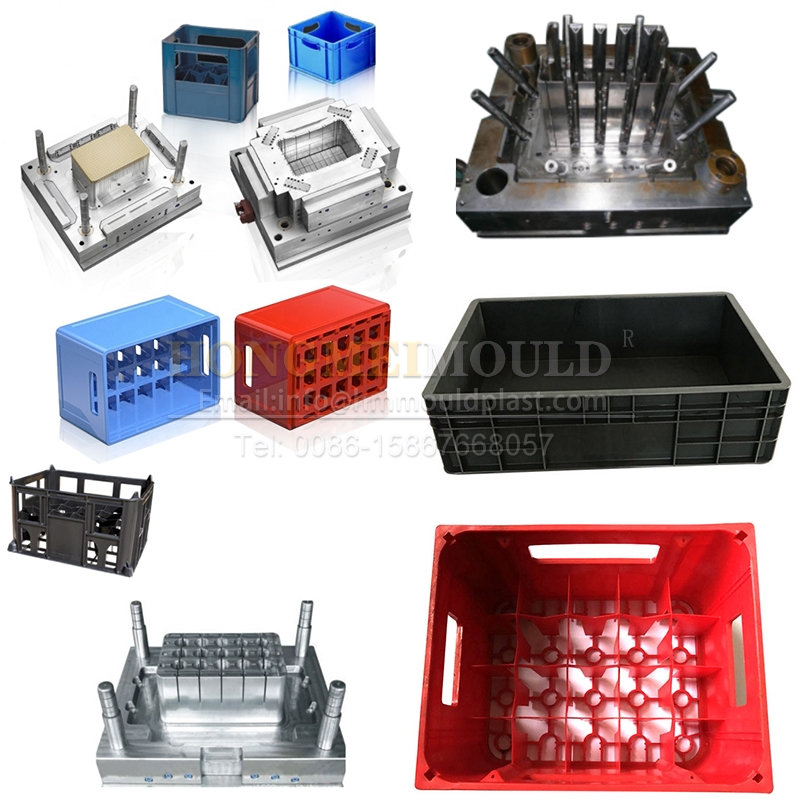The image portrays a variety of 11 distinct objects arrayed against a stark white background, making their colors—dark blue, light blue, grey, silver, red, and black—vividly stand out. Starting from the bottom right and moving left, it features an old red milk crate. Adjacent to it is a silvery, square device with four rods protruding from its sides. Above this is another crate, grey in color, likely a converted milk crate, flanked by a blue box and a red box suitable for stacking. On the far right, there's a large, rectangular, black crate. Above the crate is an object reminiscent of something a Cyberman might wear, likely a metal structure with a complex arrangement of pipes and prongs. Moving leftward, there's another set of metal devices, described as being silver and square, one featuring a prongy design and the other having a central hole. Near the top left corner, there's a small grey milk crate and a tiny blue one beside it. The scene also includes a subtle watermark that reads "M-O-U-L-D" with an accompanying telephone number, reinforcing that these items might be containers or machine parts sourced from plastic.com.